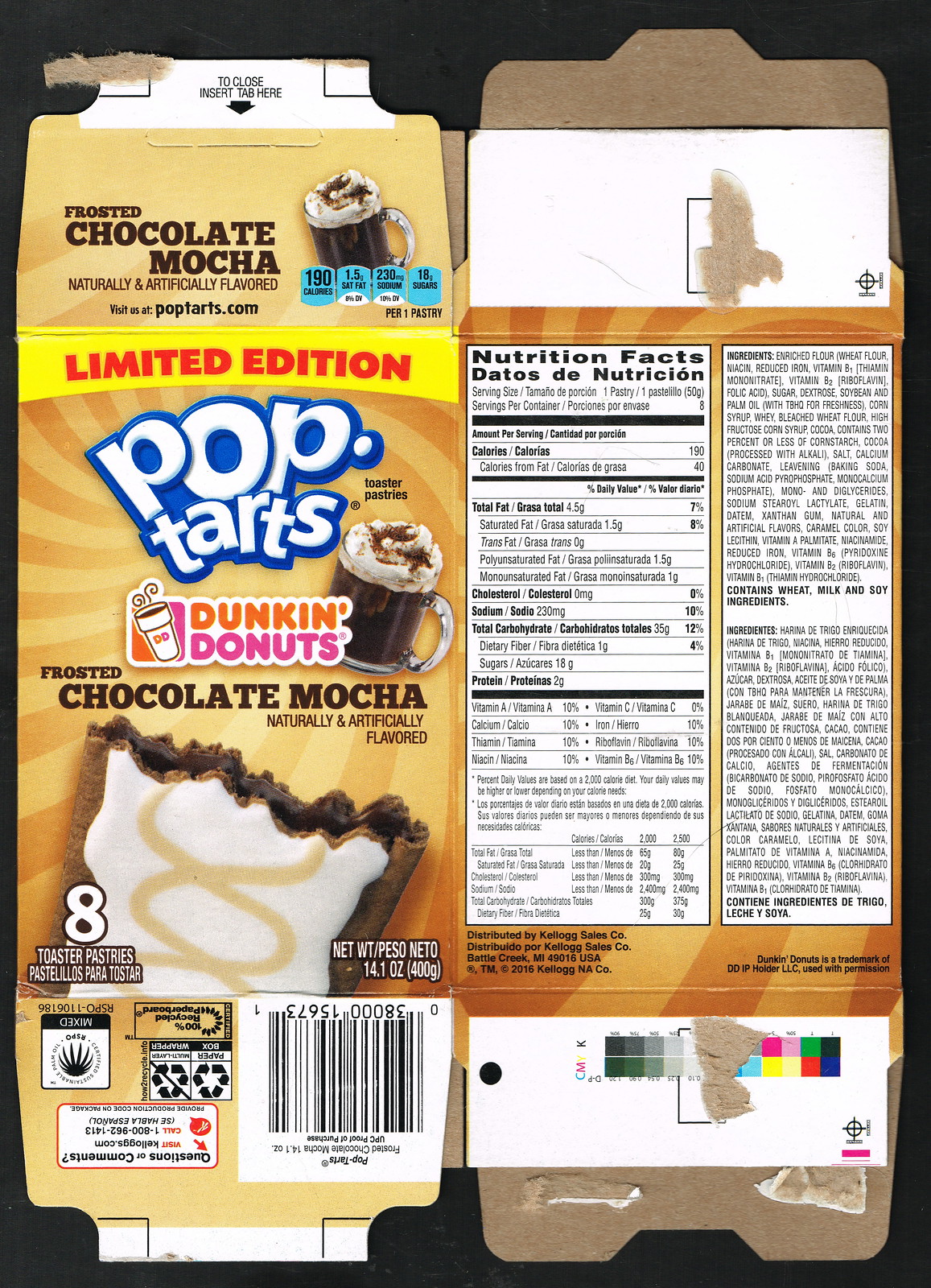The image displays a fully opened and flattened Pop-Tart box, showcasing both front and back sides, as well as one of the box's sides. The featured flavor is Frosted Chocolate Mocha, created in collaboration with Dunkin' Donuts. The front of the box prominently displays an appetizing illustration of a Frosted Chocolate Mocha Pop-Tart, designed to mirror the appearance of a Dunkin' Donuts mocha drink. The Pop-Tart has a light brown drizzle over a white frosted area. To the right of the Dunkin' Donuts logo, there's a small image of a chocolate mocha drink. Additionally, the side of the box presents Nutrition Facts, serving size information, and a barcode at the bottom. The entire image is set against a black background, making the Pop-Tart box the focal point.